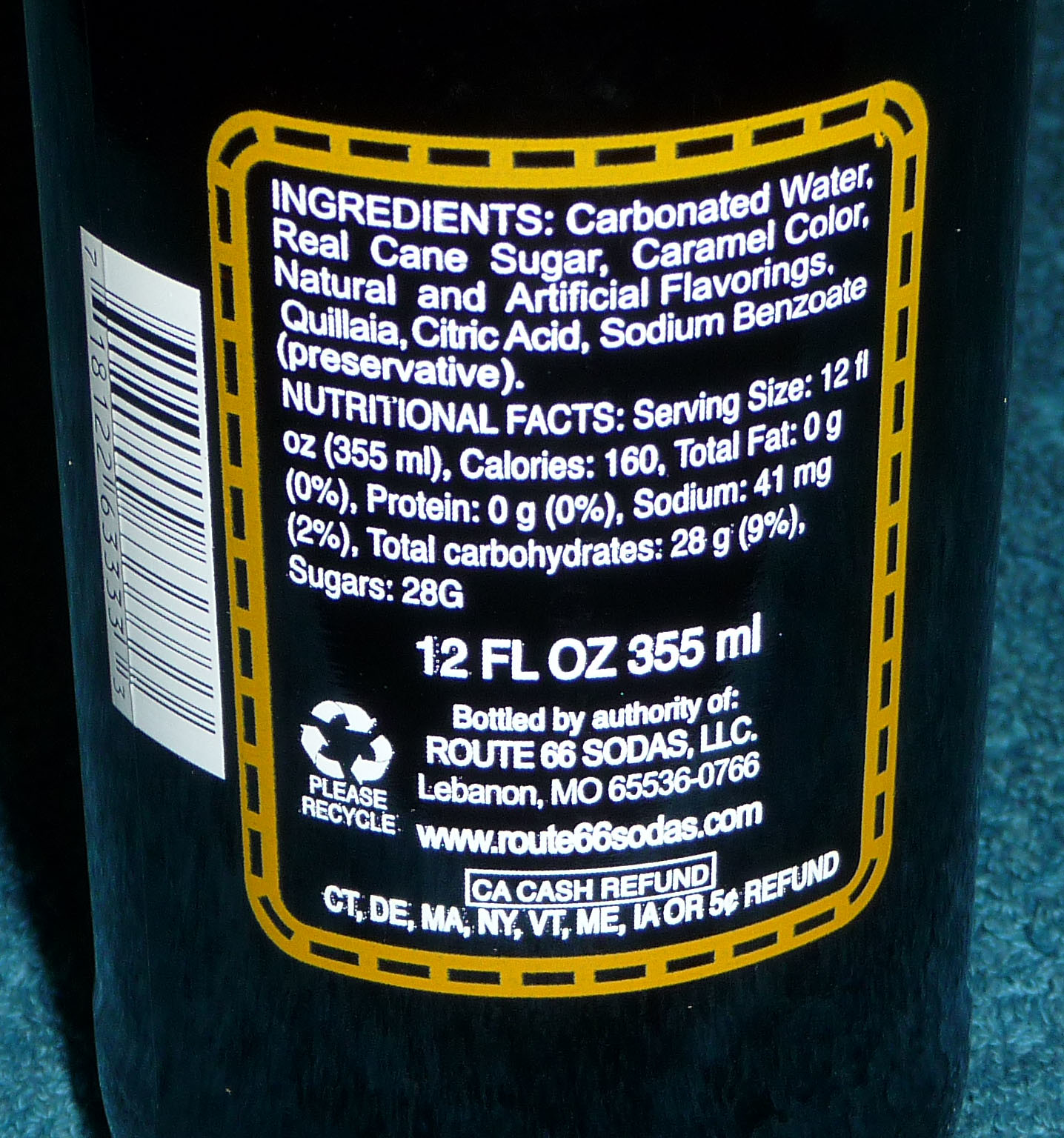This image features an extreme close-up of the back label of a black bottle, presumably a soda. The photograph does not reveal much about the surrounding environment, but a bluish surface can be seen, which could be a tabletop or carpet. Prominently displayed is a rectangular, yellowish-gold bordered ingredients label adjacent to a vertically aligned barcode. The ingredients include carbonated water, real cane sugar, caramel color, natural and artificial flavorings, Kaliya, citric acid, and sodium benzoate, a preservative. The nutritional information states a serving size of 12 fluid ounces (355 milliliters), with 160 calories, 0 grams of fat, 0 grams of protein, 41 milligrams of sodium (2% DV), and 28 grams of sugars. Also visible are the "please recycle" logo with triangular arrows, and a note that the product is bottled by the authority of Route 66 Sodas, LLC, based in Lebanon, MO 65536, with a reference to their website www.route66sodas.com and a mention of a CA cash refund offer.